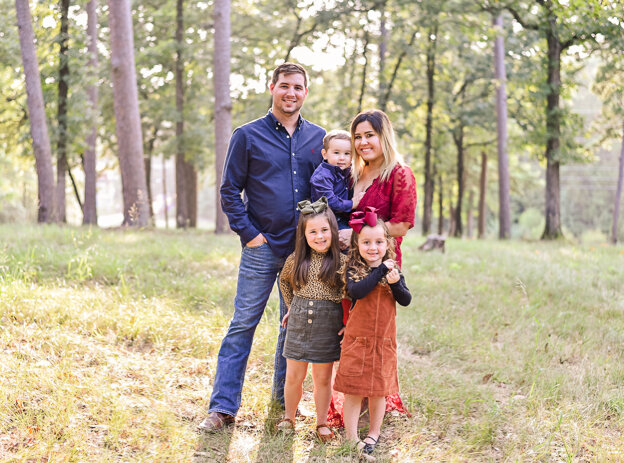An outdoor family photograph captures a beautiful Caucasian family, all smiling warmly at the camera. The dad is dressed in a long-sleeved blue button-down shirt with a collar, blue jeans, and brown boots. Next to him stands a young girl with long brown hair, wearing a gray skirt, a patterned top, brown shoes, and a red ribbon in her hair. On the right is another young girl, this one with curly, orangish-colored hair, adorned with a red ribbon, dressed in a jumper over a blue top, and wearing gray shoes. The mom, elegantly dressed in a maroon-pinkish dress, holds a cute little baby boy who is wearing a blue shirt. In the front, the young children stand close, with the girl on the left sporting brown hair and a gray skirt, while the girl on the right has curly orangish hair and wears a blue top and jumper. Both girls have ribbons in their hair. The happy family is clearly enjoying their time together outdoors.